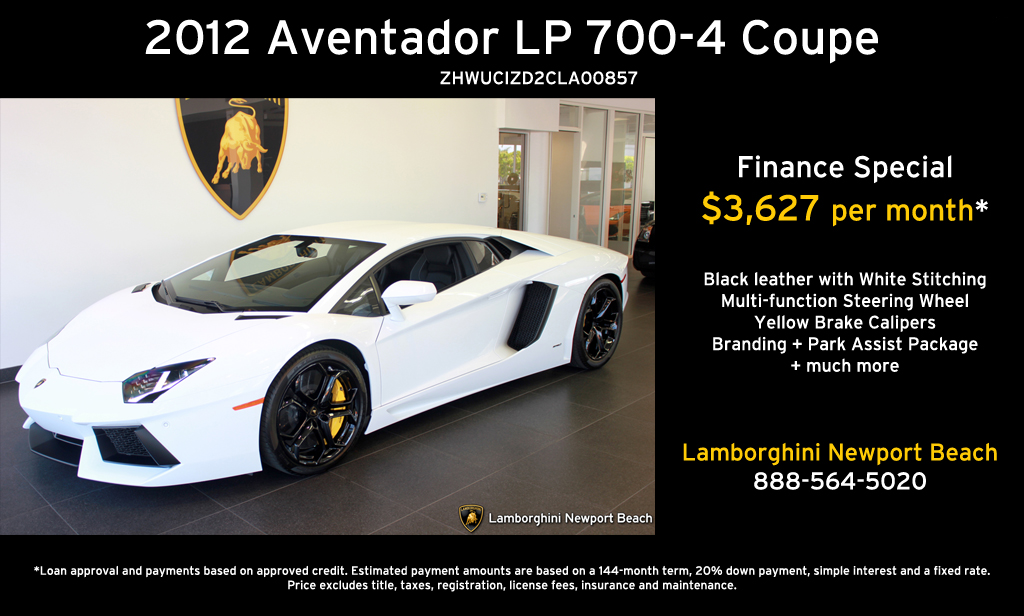This advertisement features a pristine white 2012 Lamborghini Aventador LP 700-4 Coupe with black wheels and striking yellow brake calipers. Showcased inside the Lamborghini Newport Beach dealership, the car's sleek design is emphasized by its luxurious black leather interior adorned with white stitching. The multifunction steering wheel and park assist package add to its allure. The sign in the background has a black backdrop with white and yellow lettering, highlighting the finance special of $3,627 per month. Additional details include comprehensive branding and more premium features. The dealership’s contact information and terms of loan approval are also prominently displayed at the bottom in white lettering.